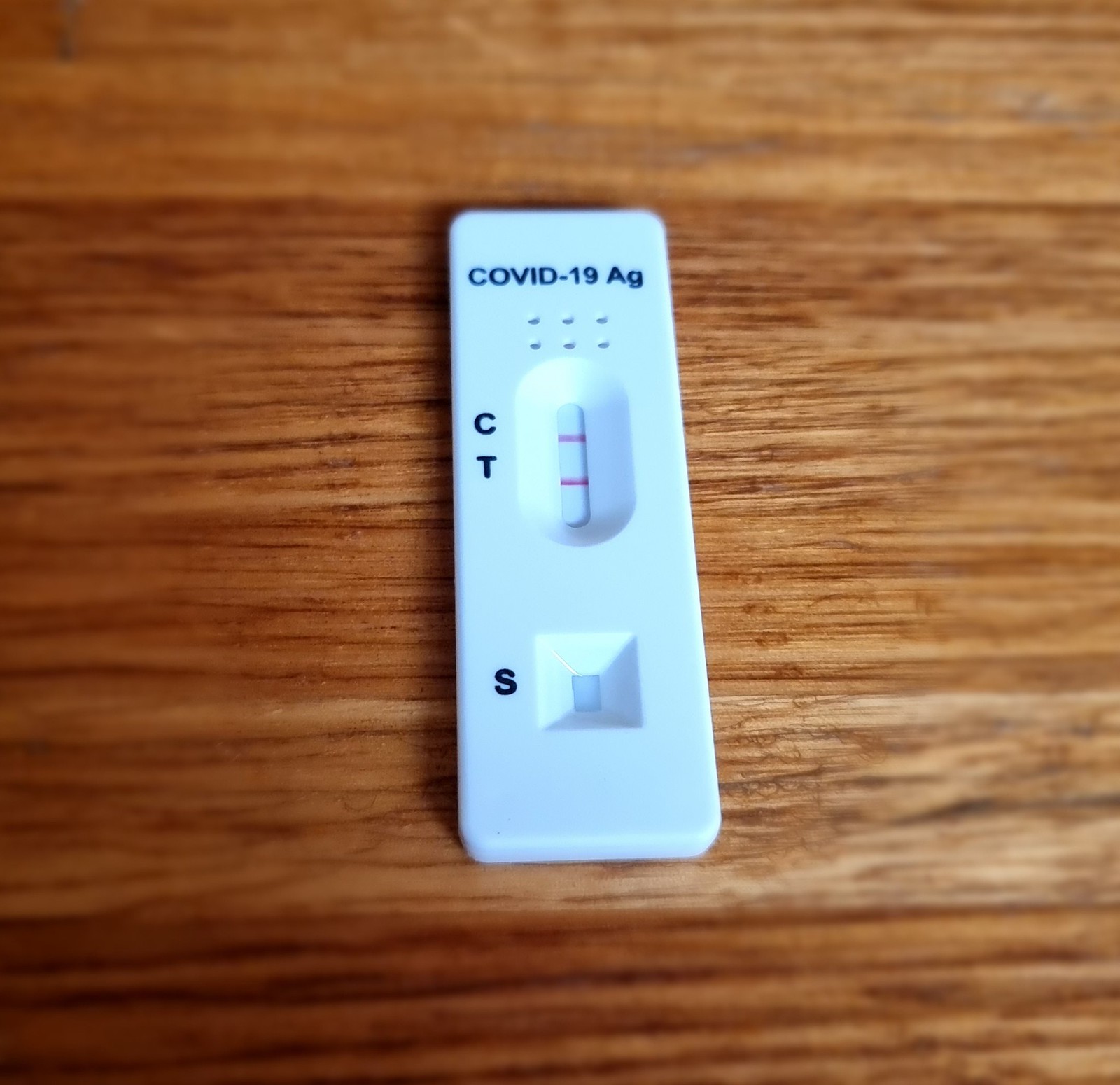The image captures a well-worn, grainy wooden table, illuminated slightly by a nearby lamp. Dominating the center of the table is a white rectangular COVID-19 antigen test, unmistakably marked with "COVID-19 AG." The test features a distinct design with an area labeled "S" at the bottom for applying the solution. Above this, there is an oval window displaying the letters "C" and "T," which indicate the test results. In this case, two red lines are visible, signifying a positive result. The test also features six small holes, likely for air ventilation. Subtle shadows cast by the light play across the surface of the test, adding depth to the scene.